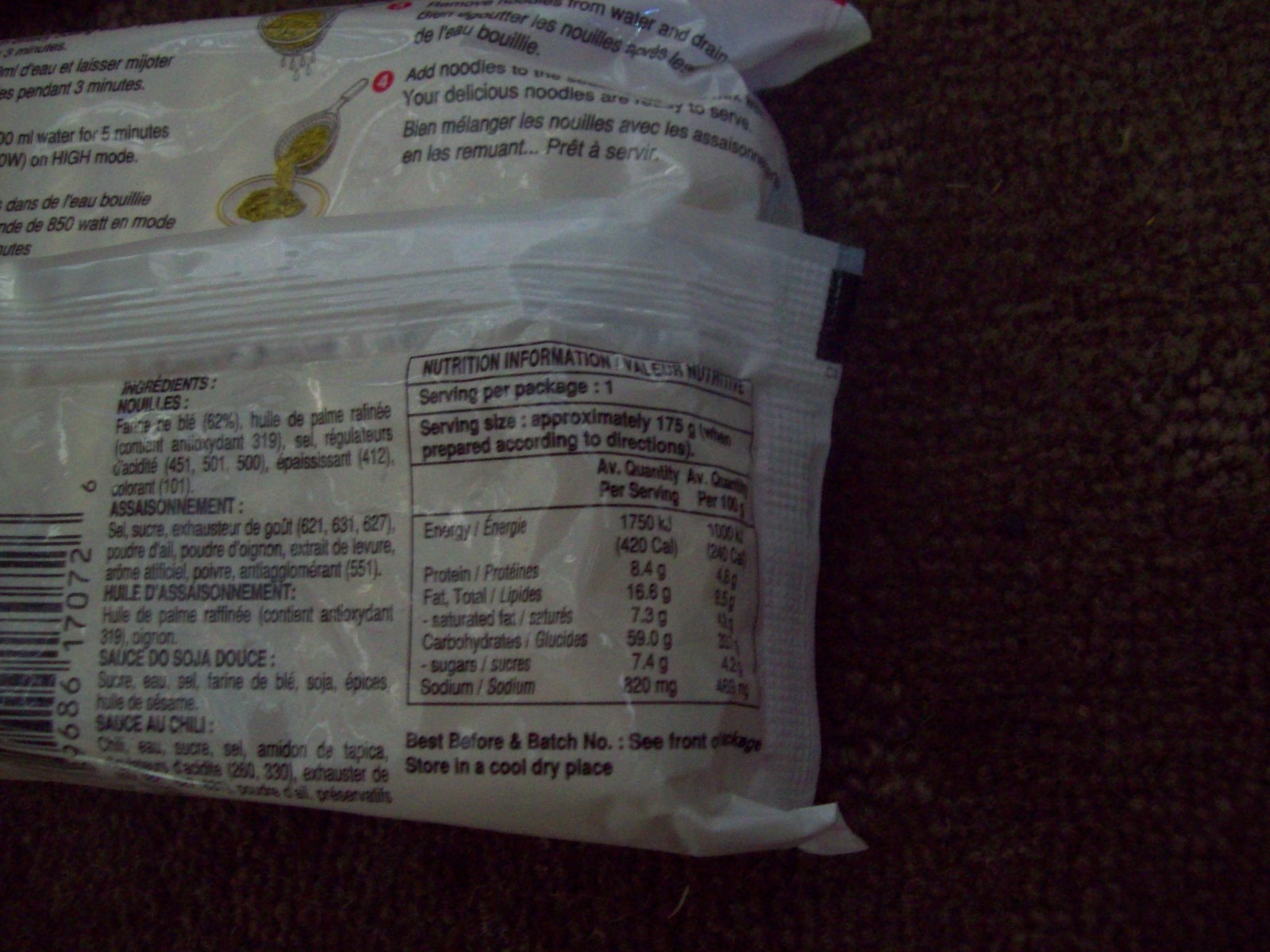A white package of ramen noodles lies on a brown carpet, showcasing various details. At the top of the package are instructions in English for cooking the noodles, while the bottom part features the same instructions in another language. A barcode is located on the left side, and the nutritional information is displayed on the right. A prominent white seam runs vertically down the middle of the package. Additionally, the package is sealed on one end. The upper section of the package shows an image of a spoon pouring noodles into a bowl. The serving size is indicated as one package, approximately 175 grams, with preparation instructions included.